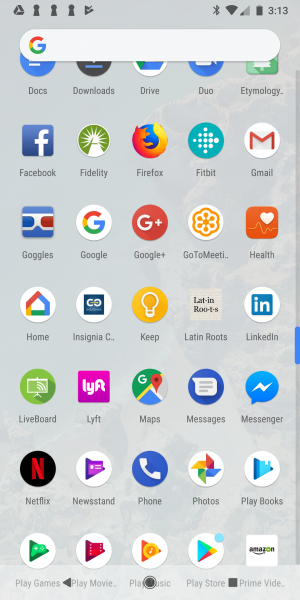This image showcases a phone screenshot depicting the home screen of an Android device. At the top left corner is a Google Drive icon followed by three dark lock symbols whose specific function is unclear. Adjacent to these is a Google Play icon. On the top right, various status icons are visible: a Bluetooth icon, a full Wi-Fi bar, a signal strength indicator showing only a quarter of full strength, a fully charged battery bar, and the time displayed as 3:13.

Prominently featured beneath these elements is a Google search bar that overlays the top row of app icons but leaves their names partially readable. The partially obscured row includes icons for Docs, Downloads, Drive, Duo, and Etymology. Below this, the next row of apps comprises Facebook, Fidelity, Firefox, Fitbit, and Gmail. Continuing downward, the subsequent row features Google, Google Plus, Google Meet (with the name truncated), and an app labeled Health. The next row showcases Home & Cigna, Keep, Latin Roots, LinkedIn, followed by three additional rows containing apps like Netflix and Newsstand.

The layout reflects a well-organized and app-packed home screen, indicative of a user who utilizes a variety of social media, productivity, and lifestyle applications.